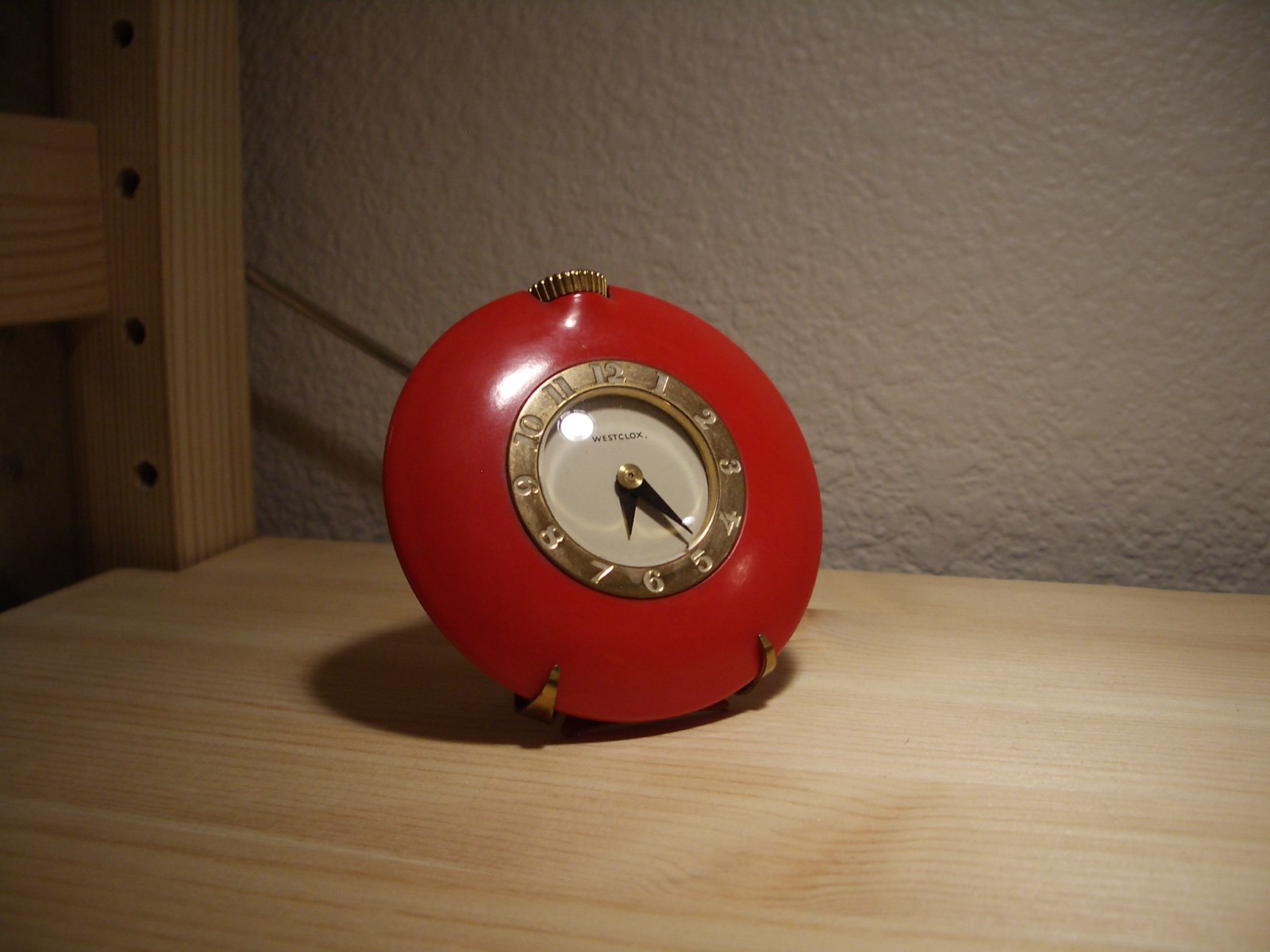A close-up photograph captures a vintage travel alarm clock in exquisite detail. The clock, circular in shape and sporting a vibrant red exterior, sits gracefully on a light-tan, beige wooden surface. Complementing the scene, the backdrop is a textured wall in a unique peachy-lilac hue, adding a touch of subtle elegance.

The clock itself is adorned with golden highlights, featuring intricate gold ribbing at the top and supported by two small gold brackets that hold it upright, slightly angling it back. At the center of the clock, a brass circle displays the time with traditional hands, sans any minute markers. The time reads 6:25, and the clock face proudly bears the name "Westclox" at the bottom, indicating its classic heritage.